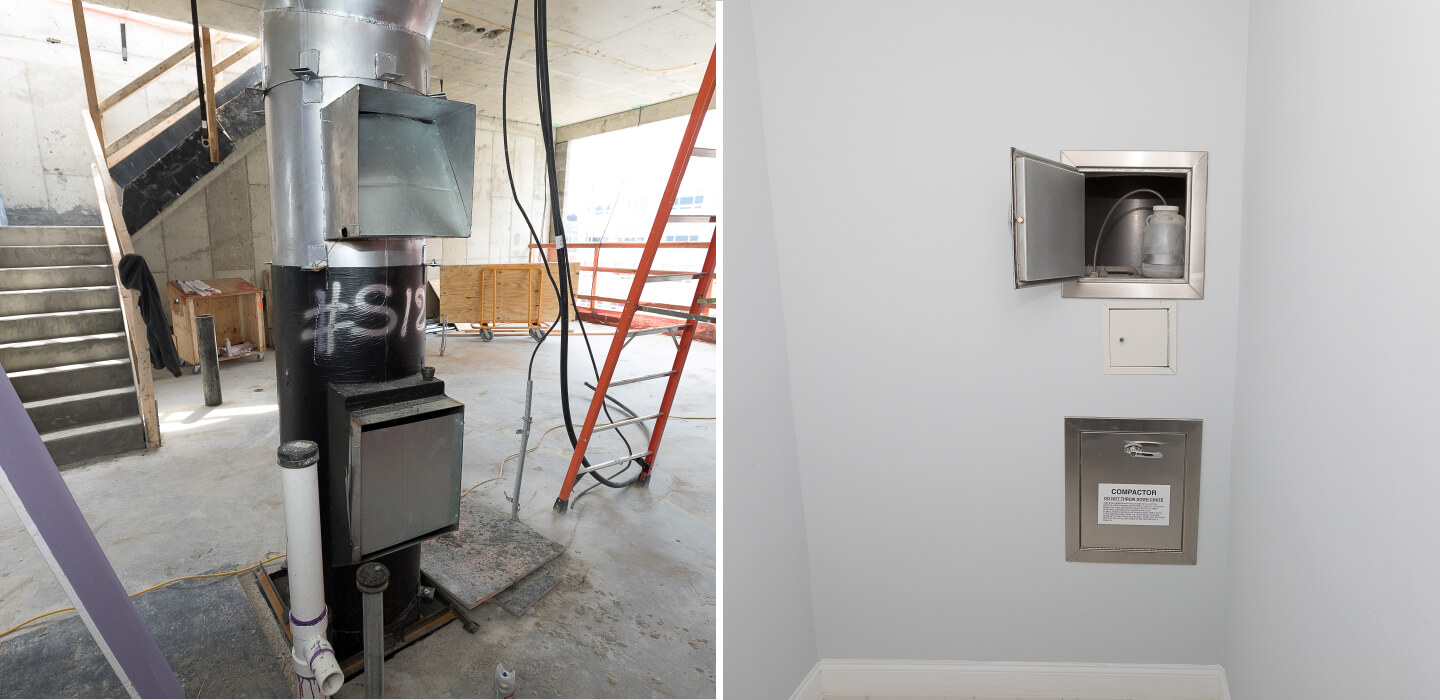This image depicts a split-view scene of a partially finished basement or lower-floor construction area, presented in two distinct segments separated by a white border. On the left side, a voluminous room features unfinished elements alongside modern touches. A prominent staircase with bare wooden handrails leads down to a finished concrete floor. Notable elements include sections of ductwork marked with "S18", an orange folding ladder leaning against the wall, and white pipes extending across the space, suggesting ongoing mechanical work. Large windows flood the area with light, enhancing the expansive feel. Wooden panels on a trolley hint at construction underway.

The right side of the image contrasts sharply with its left counterpart, showcasing a more refined space. Here, a light gray wall is punctuated by three small silver doors; one is ajar, revealing a bottle inside, while the other two remain closed. Additional fine details include a neat arrangement of what might be a mechanical container holding another vessel with a tube, adding to the technical ambiance. Black cables run through the scene, and a black hoodie hangs on the wall, contributing to the overall industrial atmosphere of this developing office or living space.